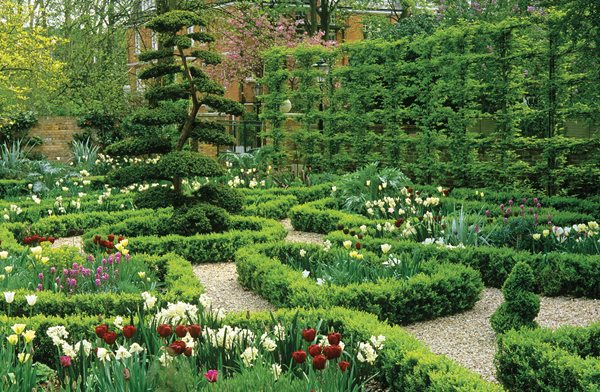This photograph showcases a meticulously landscaped public or private garden area, likely located in a city. The scene features a network of concrete or pebble paths that weave through a series of square-shaped garden plots, each bordered by carefully groomed hedges. The plots are filled with a variety of vibrant flowers, including clusters of red, white, and pink tulips, and light-colored roses, as well as some sections with purple tulips. To the right, there's a tall, grid-style trellis covered in ivy, extending about 15 to 20 feet high. A notable structure in the background is a square-shaped, three to four-story orange brick building, which might belong to a college or university. The garden is dotted with assorted shrubs and a few trees, creating a lush, inviting environment perfect for leisurely walks and plant admiration.